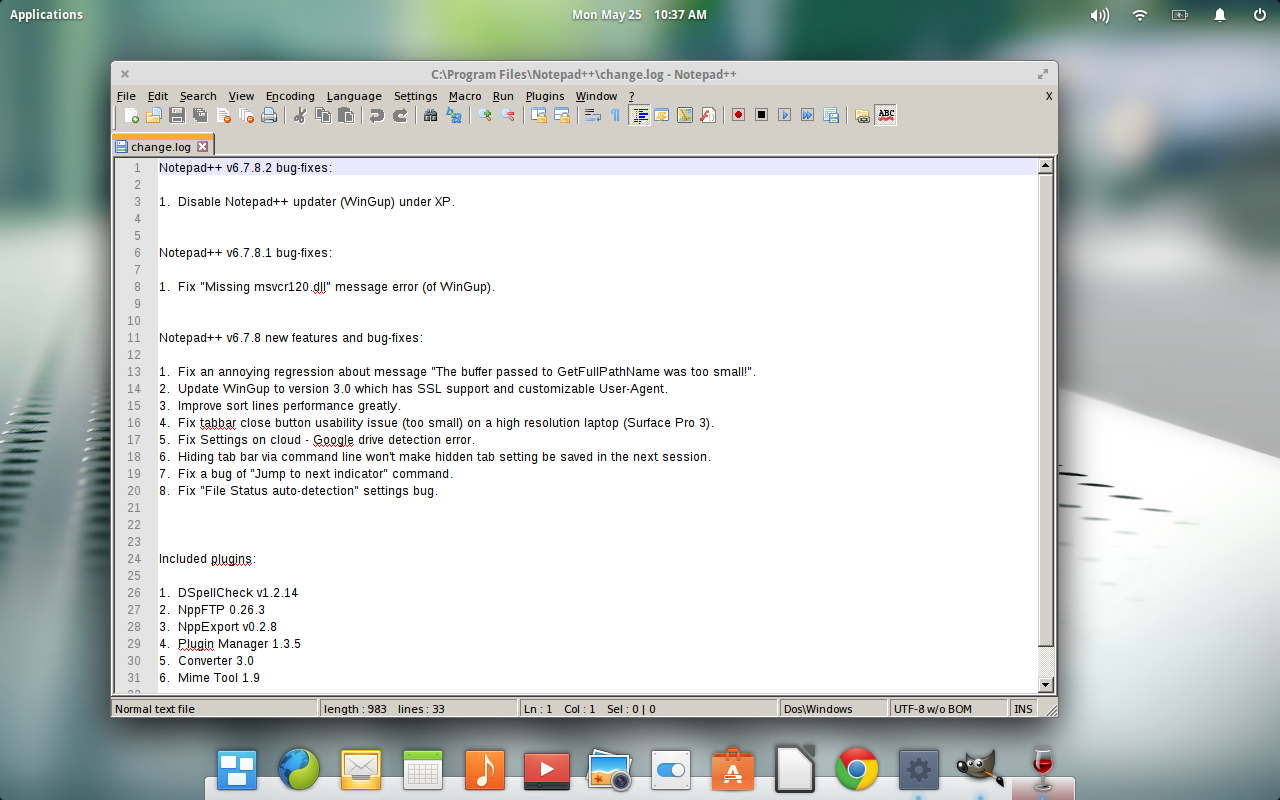The image depicts a detailed screenshot from a MacBook displaying an open Notepad application window with a changelog document. The top of the screen shows the menu bar with the word "Applications" on the left and the date and time as "MON May 25 10:37 a.m." in the center. To the right are various system icons including volume, internet connection, battery, notification bell, and power icons. The Notepad window is titled "Program Files Notepad Change Log Notepad," featuring numerous lines of text, starting with an entry labeled "1. Disable Notepad Plus Updater" followed by "Notepad 6.701 bug fixes." The changelog document is filled with information about various features, bugs, and updates relevant to Notepad. At the bottom of the screen, a dock with multiple icons is visible, including Google Chrome (a circle with red, green, and yellow colors and a blue center), GIMP, a music icon, a wine glass, and others like a yin-yang symbol and a dog.